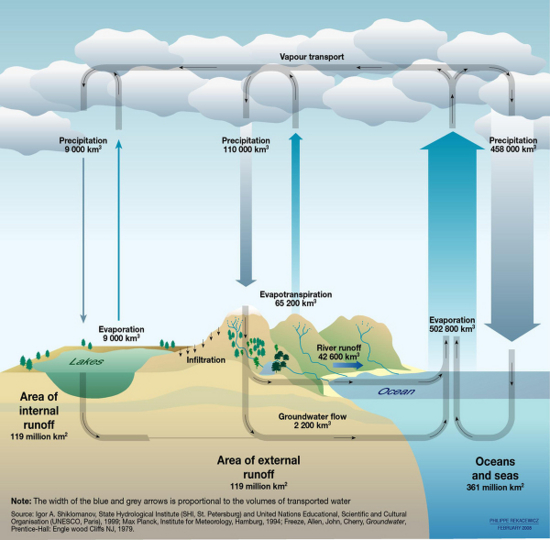This detailed square-shaped diagram, likely from a book, paper, or magazine, illustrates the process of evaporation treatment with a blue sky background transitioning to tan brown land and blue oceans and seas. At the top, clouds and arrows indicate "vapor transport," showing the movement of precipitation and evaporation. The first segment highlights "precipitation 9,000 km" and "evaporation 9,000 km," depicted above lakes. The second segment shows "precipitation 110,000 km" and "evaporation and transpiration 65,200 km," illustrated above river runoff and ground flow. The final segment details "evaporation 502,800 km" and "precipitation 456,000 km," above oceans and seas. The diagram also includes labels for areas of internal and external runoff, with various arrows and small black text explaining groundwater flow and other processes, effectively demonstrating the water cycle's movement from land to sky and back.